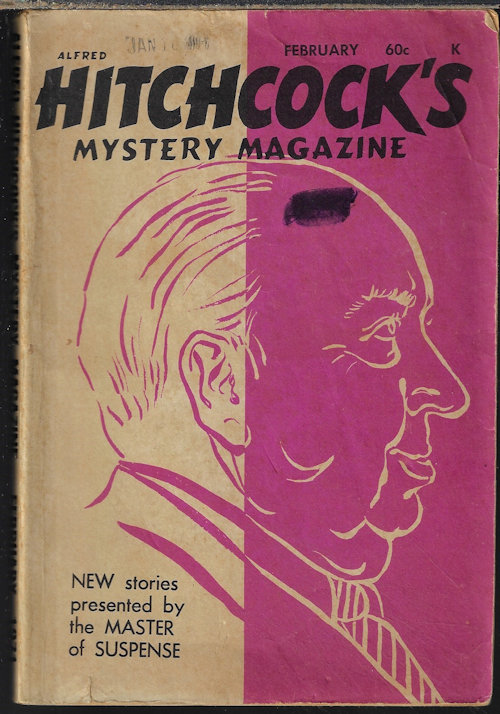The image depicts the cover of an old magazine titled "Alfred Hitchcock's Mystery Magazine." Dominated by contrasting colors, the right side of the cover is bright pink while the left side is tan. Prominently featured is a profile illustration of Alfred Hitchcock, with the right side of his head colored magenta and the left side in a light beige hue. His ear is beige, whereas his eyes, nose, mouth, and cheeks are entirely magenta. At the top of the cover, next to a mysterious 'K,' it states "Alfred Hitchcock's Mystery Magazine February" followed by the price, "60 cents." The cover also bears a partial, unreadable library stamp indicating January. At the bottom, in black font with some capitalized words for emphasis, it declares, "NEW STORIES presented by the Master of Suspense." Additionally, there is a black mark visible at the top part of Hitchcock's head, further accentuating the vintage and worn nature of this intriguing publication.